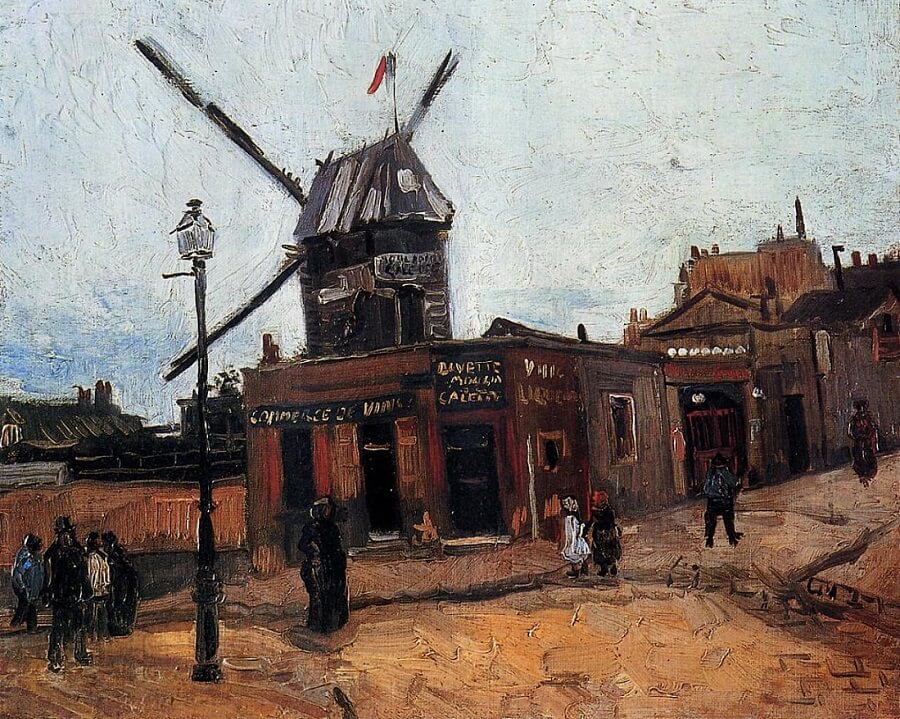The painting depicts a quaint, historical town scene characterized by a prominent windmill with large, visible blades slightly turned away from the viewer. The composition of the painting showcases a range of architectural elements, including several storefronts and houses constructed primarily from wood, with brown hues dominating both the buildings and the ground surface. The sky, painted in a mix of blue with white and grey brush strokes, adds a dynamic backdrop to the scene.

A tall, black street lamp with a glass-encased light is situated near the windmill, providing a touch of period detail. To the far right, there's what appears to be the top of a castle or a similarly grand structure, peeking out from the background. The buildings' walls bear textual signs that are indistinct but suggest names of establishments or other signage.

The street buzzes with life as numerous people, mostly in dark-colored clothing, stroll about. Among them is a girl dressed in white and another individual with red hair. The painting, although somewhat blurry and reminiscent of an older era, effectively captures the essence of a bustling small town from a bygone time.